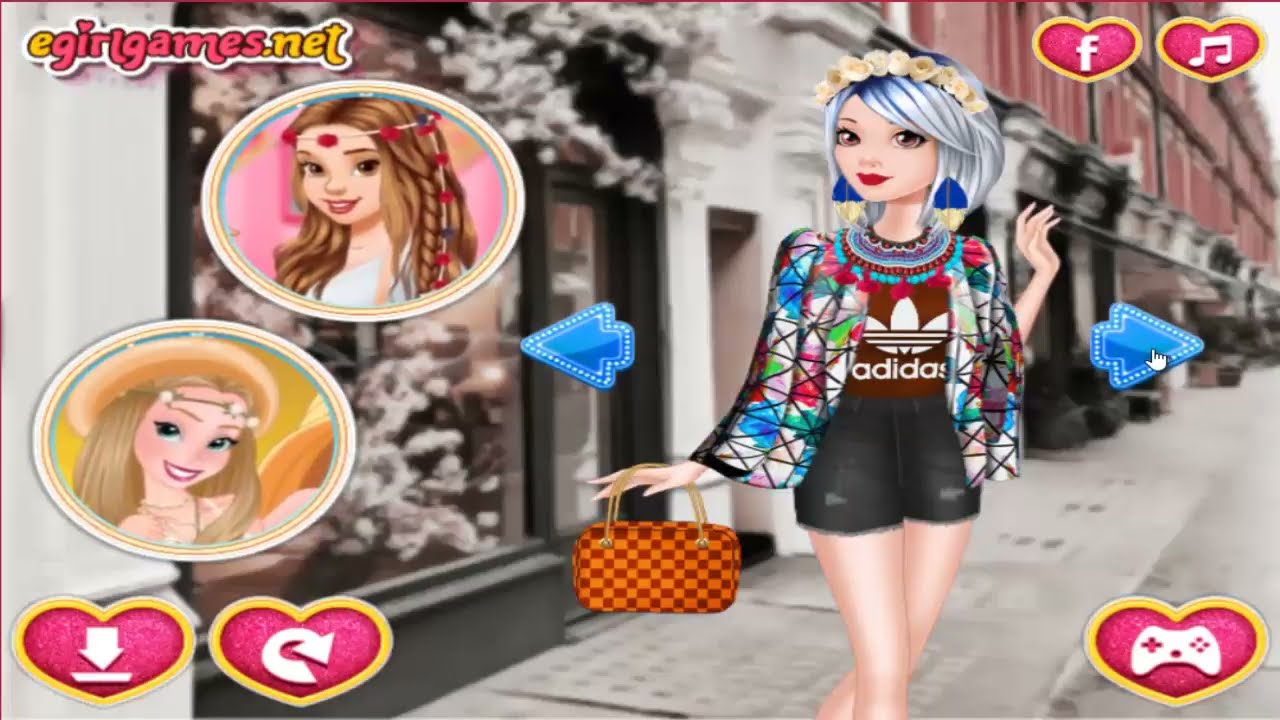In this vibrant screenshot from a video game, dominated by pastel and vivid tones, a striking female character stands slightly off-center, capturing immediate attention with her detailed and colorful ensemble. With her head turned slightly to the left but her large, brown eyes facing forward, her dark blue hair transitions seamlessly into a shimmering silver as it cascades down, partly flowing to her left. Floral and feather decorations, featuring blue on top and yellow underneath, adorn her head, complementing her bright pink lips and fully visible earrings.

She wears a brown Adidas shirt paired with short black shorts, showcasing her very light complexion. Over her shoulders, a multicolored scarf interweaves hues of red, blue, and green, adding to her eclectic fashion statement. Her right hand is raised, fingers pointing upward, while her left hand, level with her hips, holds a purse with a mix of light and dark orange colors and yellow straps, hanging off her fingertips.

Set against a serene park-like background featuring a pond, flowers, a walking path, and trees, various interactive game elements adorn the scene. In the upper right corner, two hearts house an "F" for Facebook and a musical note. The lower right corner features a heart with a game card image. In the bottom left, a heart with a down arrow and another with a refresh symbol are present, along with two circular character portraits: a female with a straw hat and light brown hair in the lower circle, and another with a bandana decorated with red dots in the upper circle.

Arrows pointing left and right flank the main character, reinforcing the navigational aspect of the game. The game's origin is marked by "egirlgames.net" displayed prominently in the upper left corner, solidifying the image as a snapshot from an interactive digital landscape designed for an engaging user experience.